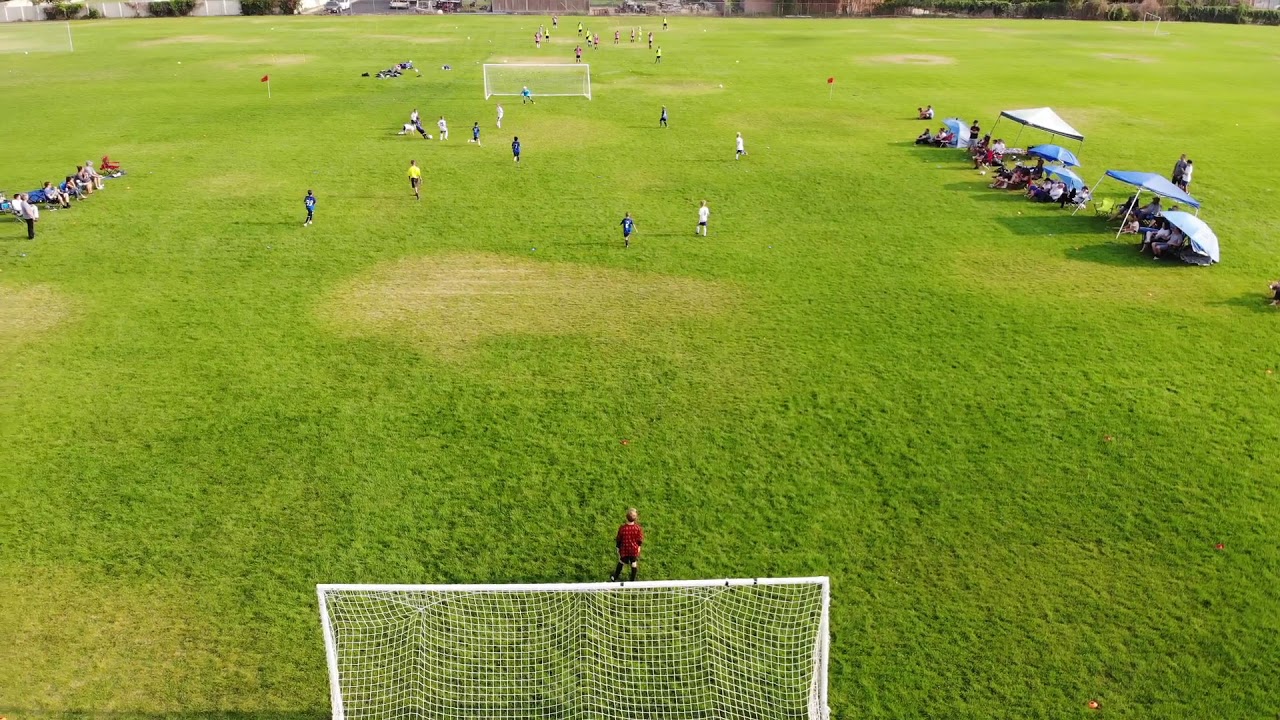The aerial image captures a lively youth soccer match from above, centered just behind one of the goals. The expansive, mostly green field features scattered brown patches, indicating it may need some maintenance. In the forefront, a young goalkeeper in a distinct red uniform stands alert in front of the white goalposts with white nets, ready to defend. Two teams are actively engaged in play, one in blue and black jerseys and the other in white jerseys, with a referee in a yellow and black shirt overseeing the match from the middle of the field. Flanking the field, parents and spectators sit comfortably under various tents and umbrellas, suggesting potential rain, as they enthusiastically support the children. In the distant background, another soccer game unfolds on an adjacent field.